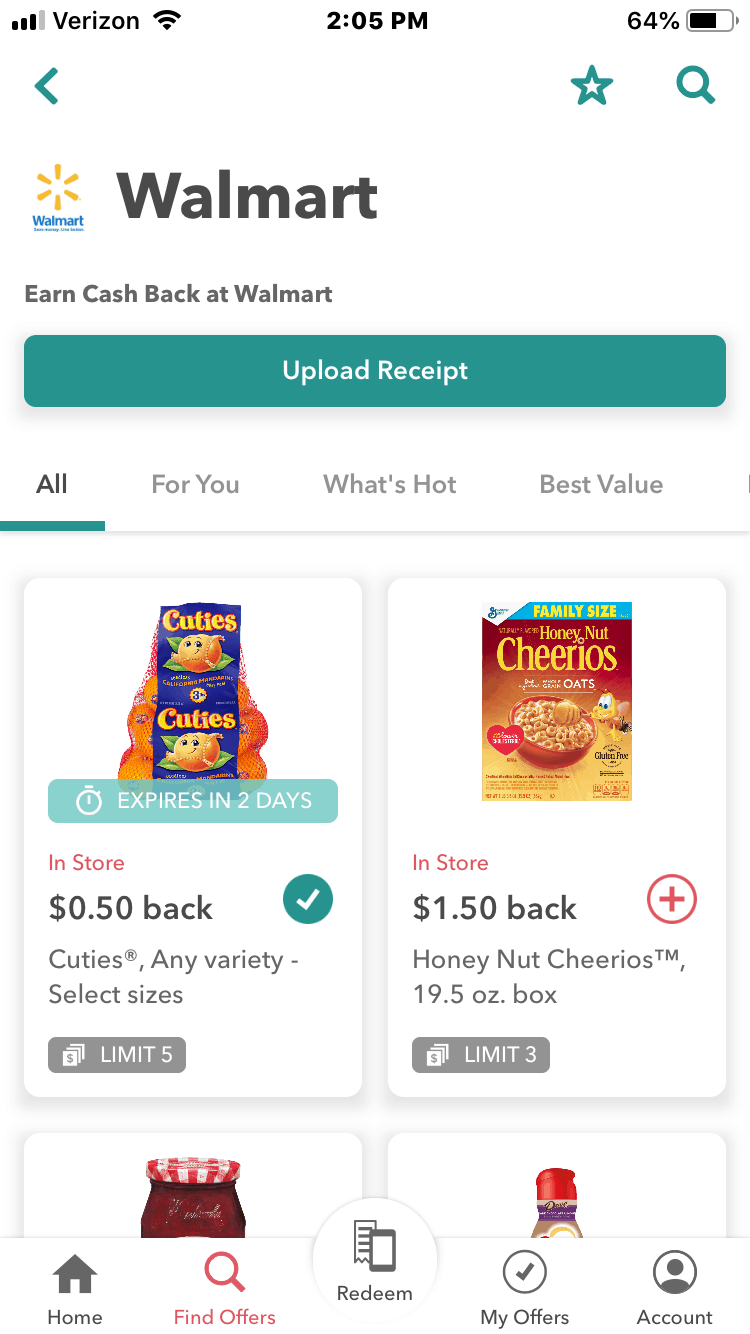The image appears to be a screenshot taken from a mobile or tablet device, featuring an app likely related to shopping rebates and offers. The specifics of the operating system are not visible. The device is connected to Verizon, displaying three out of four bars of signal strength and full Wi-Fi, while the time is 2:05 p.m., and the battery level is at 64%.

At the top left, there is a green arrow that can point either left or right. Adjacent to this are icons for favorites (a star) and search (a magnifying glass). Below these icons, the Walmart logo is prominently displayed, featuring a yellow sun or flower design with the word "Walmart" beneath it. The text "Earn Cash Back at Walmart" follows, along with a green rectangle containing the instruction "Upload Receipt" in white text.

The interface includes several categories such as "All for You," "What's Hot," and "Best Value." At the bottom navigation bar, icons are present for different sections: a house icon for "Home," a magnifying glass for "Find Offers" (highlighted in red indicating the current section), a circle depicting a receipt within a smartphone for "Redeem," a checkbox icon for "My Offers," and a person icon for "Account."

Visible offers for Walmart include:
1. A bag of Cuties oranges, expiring in two days, available in-store with a cash back offer of 50 cents. The offer is marked as selected, specifying any variety of Cuties, select sizes, with a limit of five.
2. A family-size box of Honey Nut Cheerios, with an in-store offer of $1.50 cash back. This offer is not yet selected, specifying a 19.5-ounce box with a limit of three.

Two additional items partially visible are identified as a jar of Welch's strawberry spread and a bottle of Coffee-mate syrup, though details of their offers are not fully discernible.

Overall, this screenshot illustrates the various cash back offers available for Walmart shoppers through this rebate app.